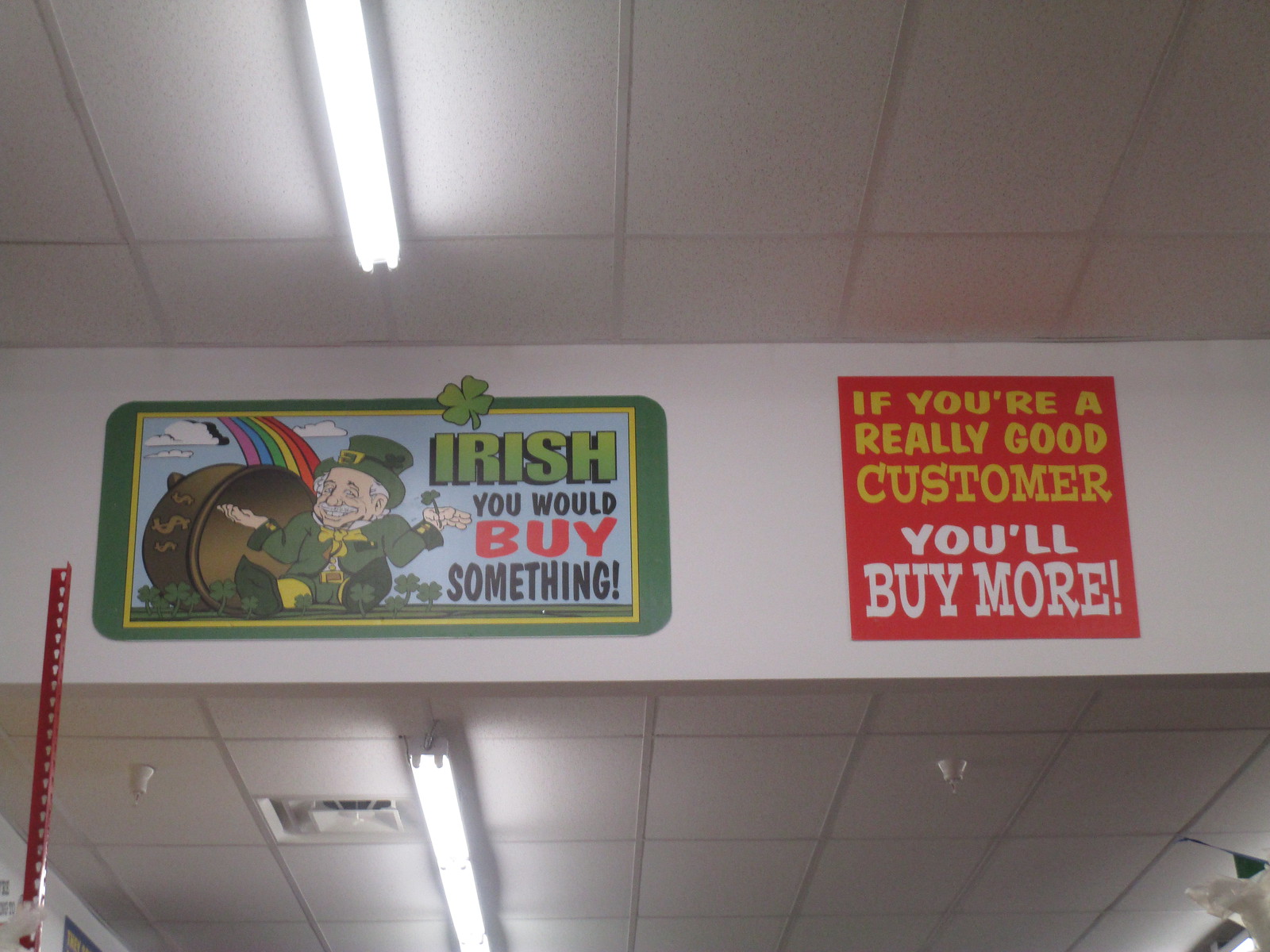In a store with a drop tile ceiling and bright white fluorescent lighting, we see two distinct signs displayed against a white-painted soffit. To the right, near the ceiling, hangs a red bag-holding apparatus with various hooks.

The first sign, on the right, features a whimsical St. Patrick's Day theme. A cheerful, green-outfitted leprechaun with white hair and a mustache sits cross-legged in front of an upturned pot of gold at the end of a rainbow. The blue sky and white clouds in the background complement the vivid green and yellow trim of the sign. Atop the sign, a shamrock adds an extra touch of festivity. The message on the sign reads, "Irish you would buy something," with "Irish" in green, "you would" and "something" in black, and "buy" in red. The leprechaun, holding a shamrock in his left hand, has his right hand extended toward the now-empty pot of gold.

The second sign, to the left of the leprechaun sign, is bold and eye-catching with a red background and yellow and white text. The top section in yellow reads, "If you're a really good customer," followed by "you'll buy more" in white text.

Additional details include the partial view of drop tiles and a fluorescent light fixture in the ceiling. The store's ceiling area also features a smoke detector and a sprinkler system, adding to the practical aspects of the described scene.